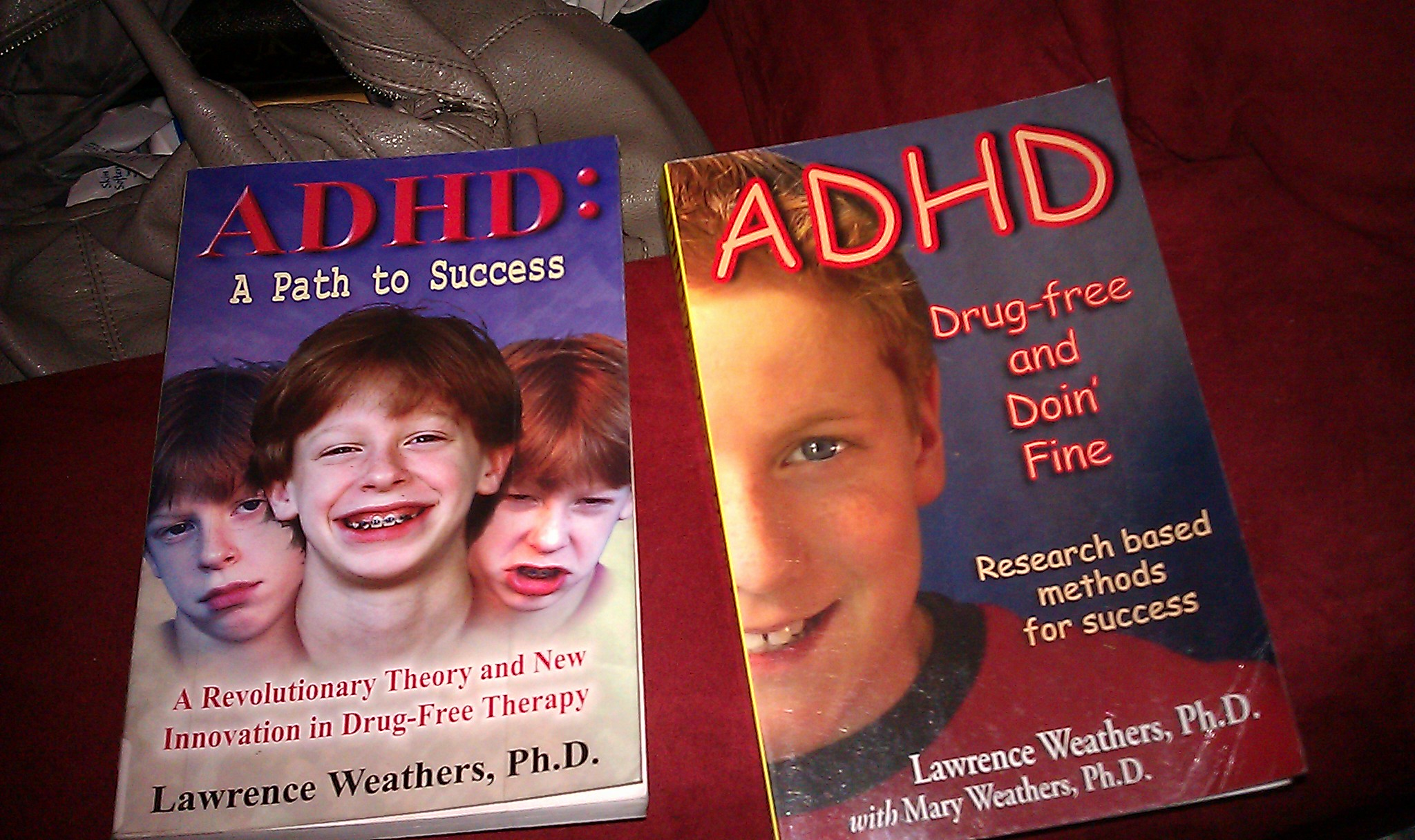In the photograph, two books are laid on a red, fabric-covered table. The book on the left has a blue background and features the title "ADHD: A Path to Success" in red text, with the subtitle "A Revolutionary Theory and New Innovation in Drug Therapy" prominently displayed in red text below. The cover showcases three images of the same redheaded child, each depicting different emotions: despondent in the center, smiling on the left, and looking angry or disgusted on the right. The author's name, Lawrence Weathers, PhD, is displayed in black text at the bottom.

To the right, the second book also has a blue background. Its title, "ADHD: Drug-Free and Doing Fine," is in bold white text with red borders. Below, in yellow text, is the subtitle, "Research-Based Methods for Success." The bottom of the cover reveals the authors: Lawrence Weathers, PhD, and Mary Weathers, PhD. This book features an image of a smiling child, specifically the right half of his face.

Both covers highlight a treatment approach to ADHD, emphasizing success and innovation, with a clear focus on the child-centered aspect of therapy.